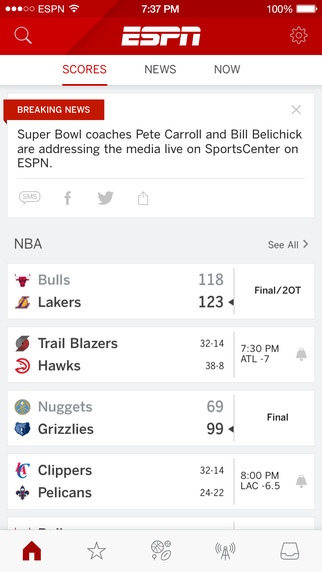Detailed Caption:

The image showcases the ESPN app being viewed on a mobile device, evident from its vertical orientation. At the top of the screen, a status bar displays three out of five white dots indicating signal strength, along with the Wi-Fi icon, the time reading 7:37 p.m., and a full 100% battery charge. The ESPN logo is prominently featured in white at the top center.

Towards the upper section of the screen, a gray-colored magnifying glass icon on the left denotes the search function, while a gray cogwheel on the upper right represents the settings option. Below these icons, a white border houses the navigation menu with "Scores" highlighted and underlined in red, indicating it is the active section, along with other options such as "News" and "Now".

Underneath the navigation menu, a breaking news headline is prominently displayed, stating, "Super Bowl coaches Pete Carroll and Bill Belichick are addressing the media live on SportsCenter ESPN." This headline is accompanied by share and interaction icons for SMS, Facebook, Twitter, and a download option.

Further down, an "NBA" section is visible with a "See All" option for more detailed information. The current game scores listed include:
- Bulls 118 vs. Lakers 123 (final after two overtimes)
- Trailblazers 32 vs. Hawks 38 (in progress: 14 for Trailblazers, 8 for Hawks)
- Nuggets 69 vs. Grizzlies 99 (final score)
- Clippers 32 vs. Pelicans 24 (in progress: 22 for Pelicans)

At the very bottom of the screen, there is a navigation bar with icons representing Home, Favorites, Sports, Broadcast, and possibly a Download option.

Overall, the image provides a comprehensive view of the ESPN app interface on a mobile device, complete with live updates and various interactive options.